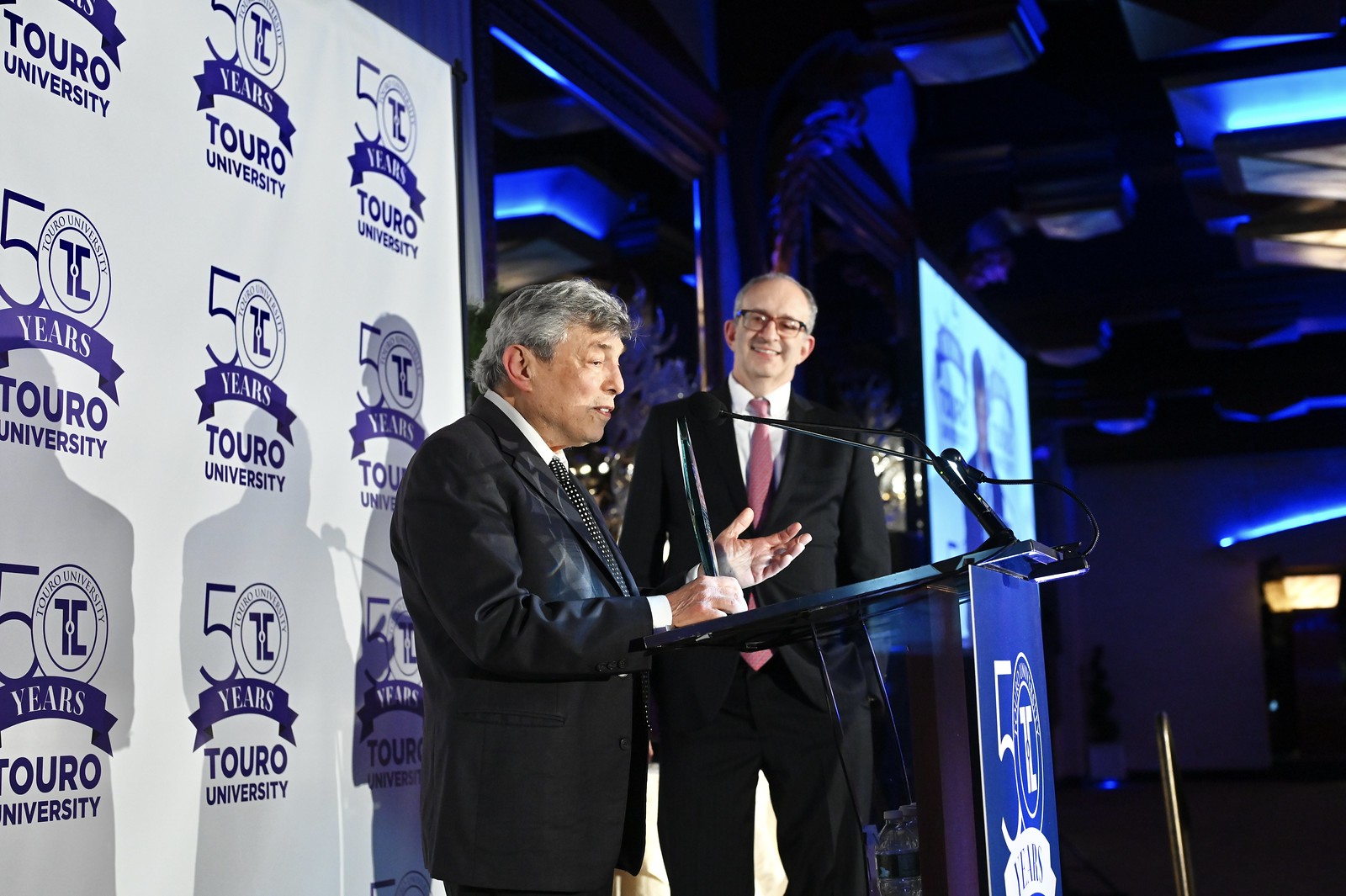In the photograph, two older gentlemen are standing on a stage adorned with a large white backdrop that reads "50 years Touro University," featuring the university's logo in place of the zero. The focus is on an older man, likely in his late 50s or early 60s, positioned just left of center at a podium, speaking into a microphone. He has gray hair and is attired in a black suit coat, a white button-down shirt, and a black tie with white polka dots. In his right hand, he holds a black award, resting it on the podium, while he gesticulates with his left hand. Beside him, to the right in the background, stands another man of a similar age, possibly in his 50s, with short gray hair and black-framed glasses. This second man, dressed in a black suit with a pink tie and white shirt, is smiling as he looks on at the man at the podium. The scene vividly captures a celebratory moment, possibly an award presentation, embodying a sense of pride and accomplishment.